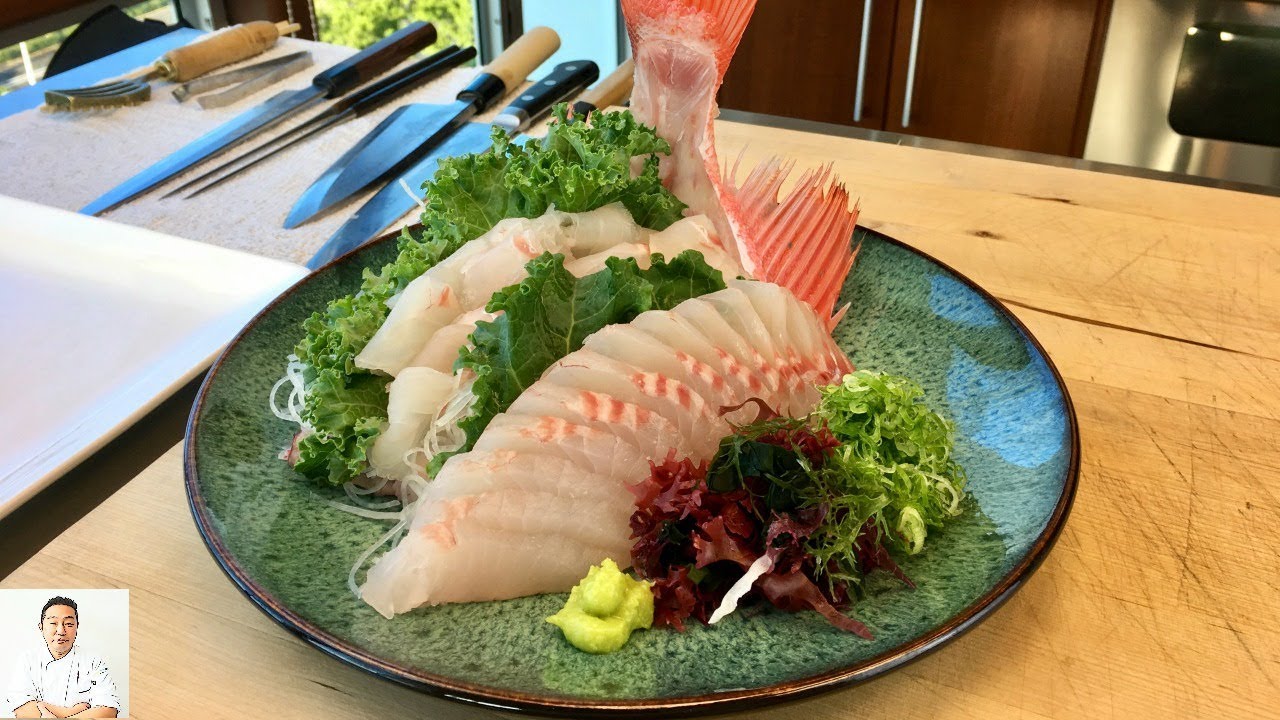This image captures a meticulously plated culinary presentation on a dark green, speckled ceramic plate with a brown edge. The plate sits on a well-worn wooden cutting board, evident from prominent knife marks, hinting at extensive use. The central focus of the plate is exquisitely sliced fish fillets, demonstrating fine knife skills. The fish skin, fins, and tail are used decoratively, creating an impressive and appetizing display. Accompanying the fish are a bed of mixed greens, including radicchio and lettuce, as well as a seaweed salad placed on the right side. A small dollop of wasabi is positioned at the front of the plate. The background reveals an array of kitchen tools, including sharpened knives, tongs, and a fork, possibly used in the preparation, placed on a countertop or prep station. In the lower left corner of the image, a photograph of a 40-ish Asian chef in a short-sleeved white jacket, arms crossed, adds a personal touch, although his name is not mentioned. The setting appears to be in front of dark brown cabinets with metal handles and an oven door.